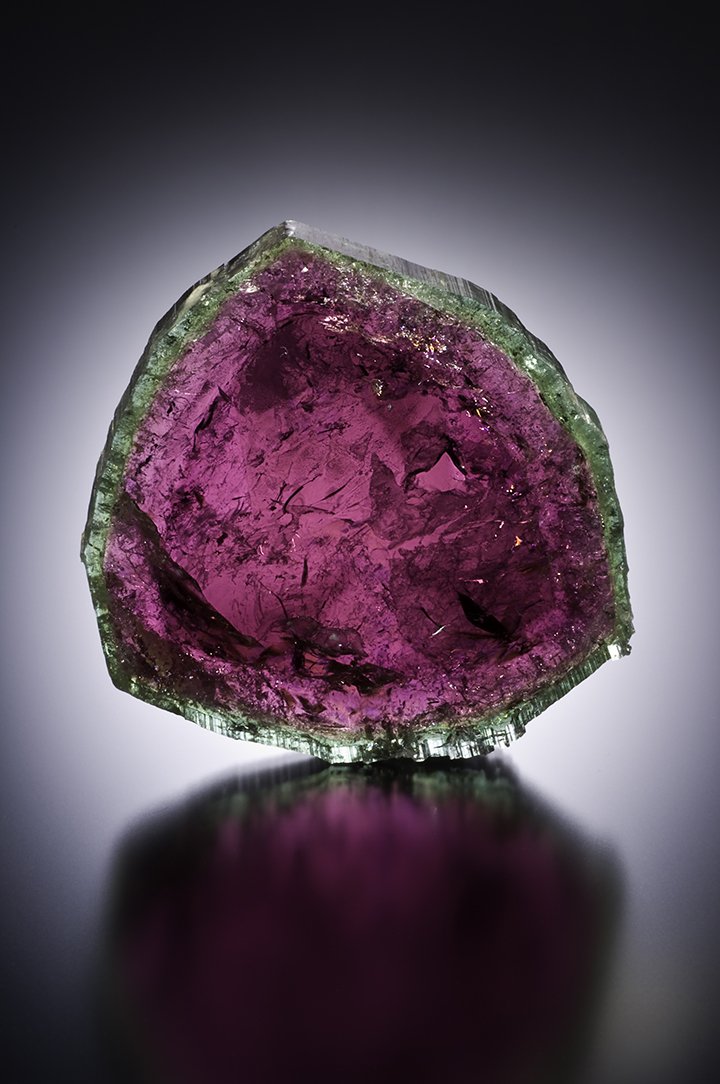The image depicts a highly detailed, close-up photograph of a split geode that resembles a vibrant and artistic gemstone. The geode's interior is predominantly a striking pink or raspberry hue, reminiscent of a dragon fruit, while its outer shell features a transparent, greenish-blue crystal. The crystalline structure appears shattered and irregular due to the way it has been broken. The stone is thin, adding to its delicate and intricate appearance. There's a notable glistening effect caused by the lighting, emphasizing the geode's shiny facets. The geode rests on a semi-gloss finished table, reflecting the stone in a coherent yet slightly surreal manner. The background is kept neutral in grey and white tones, enhancing the focus on the vivid colors of the geode. The image has a strong vignette effect and appears to be backlit, casting a mild yet clear light through the transparent portions of the stone, creating an almost ethereal glow. The photograph strikes a balance between realism and artistry, making it look slightly fantastical and highly picturesque.